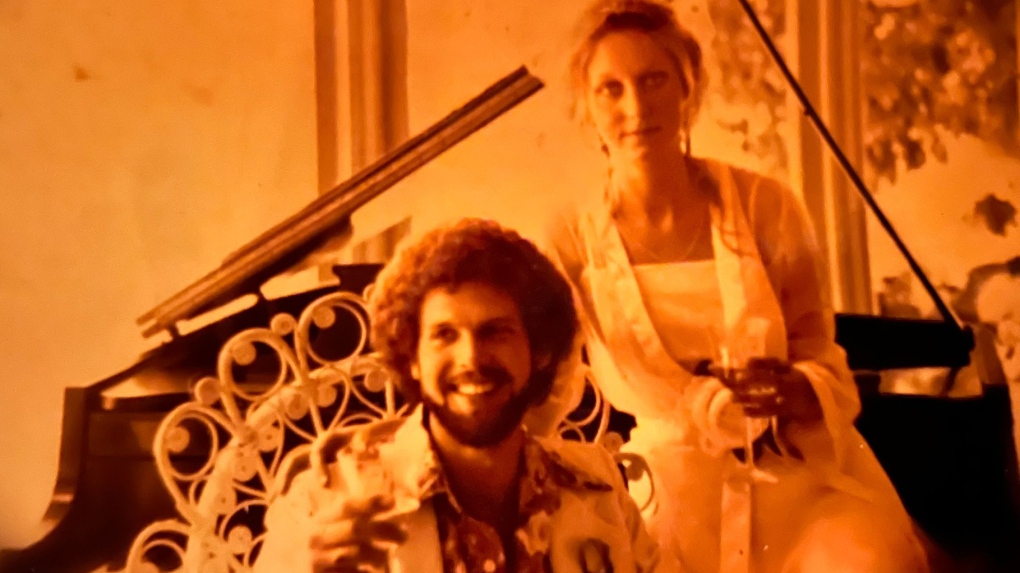The photograph is a vintage, sepia-toned image from the 1970s, capturing a man and a woman in a celebratory moment. The man, pictured from the torso up, sits on the left in a wicker chair with ornate circular patterns. He has curly brown hair styled in a bushy manner reminiscent of an afro, and sports a beard and mustache. His broad smile reveals his top teeth, and he wears a floral collared shirt under a white suit jacket. His right hand holds a glass, suggesting a toast.

To his right stands a woman with blonde hair styled in an updo, leaning against a grand piano. Her attire includes a white strapless dress with a sheer jacket over it, complete with sheer sleeves. She holds a champagne glass in her hand and gazes directly at the camera with a neutral expression. The background features an orangish wall with columns and possible tree branches or leaves extending down from the upper right corner, suggesting an indoor setting with vintage decor.